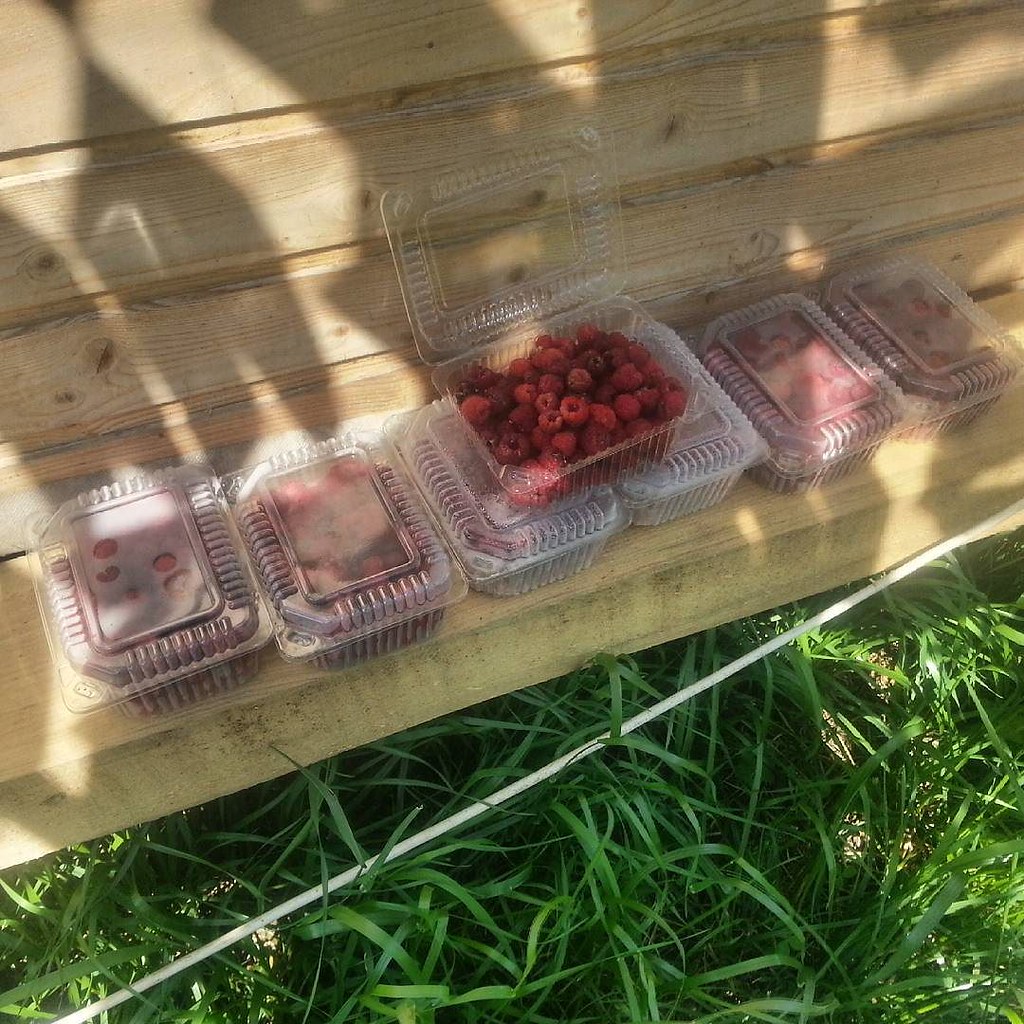The image showcases a row of six clear plastic containers, each brimming with vibrant red raspberries, neatly lined up side by side on a light-colored, beech wood bench. Notably, a seventh container sits open atop the middle two containers, revealing the detailed texture and vivid red hue of the raspberries within. The bench, composed of light wooden slats, stands above an area of lush, green grass, illuminated by sunlight that creates a dynamic play of light and shadows throughout the scene. A white string stretches diagonally from the middle right edge to the bottom left corner, casting additional shadows over the bench and the raspberry containers below. The inviting outdoor setting, possibly a park or backyard, adds a rustic charm to the display of fresh fruit.